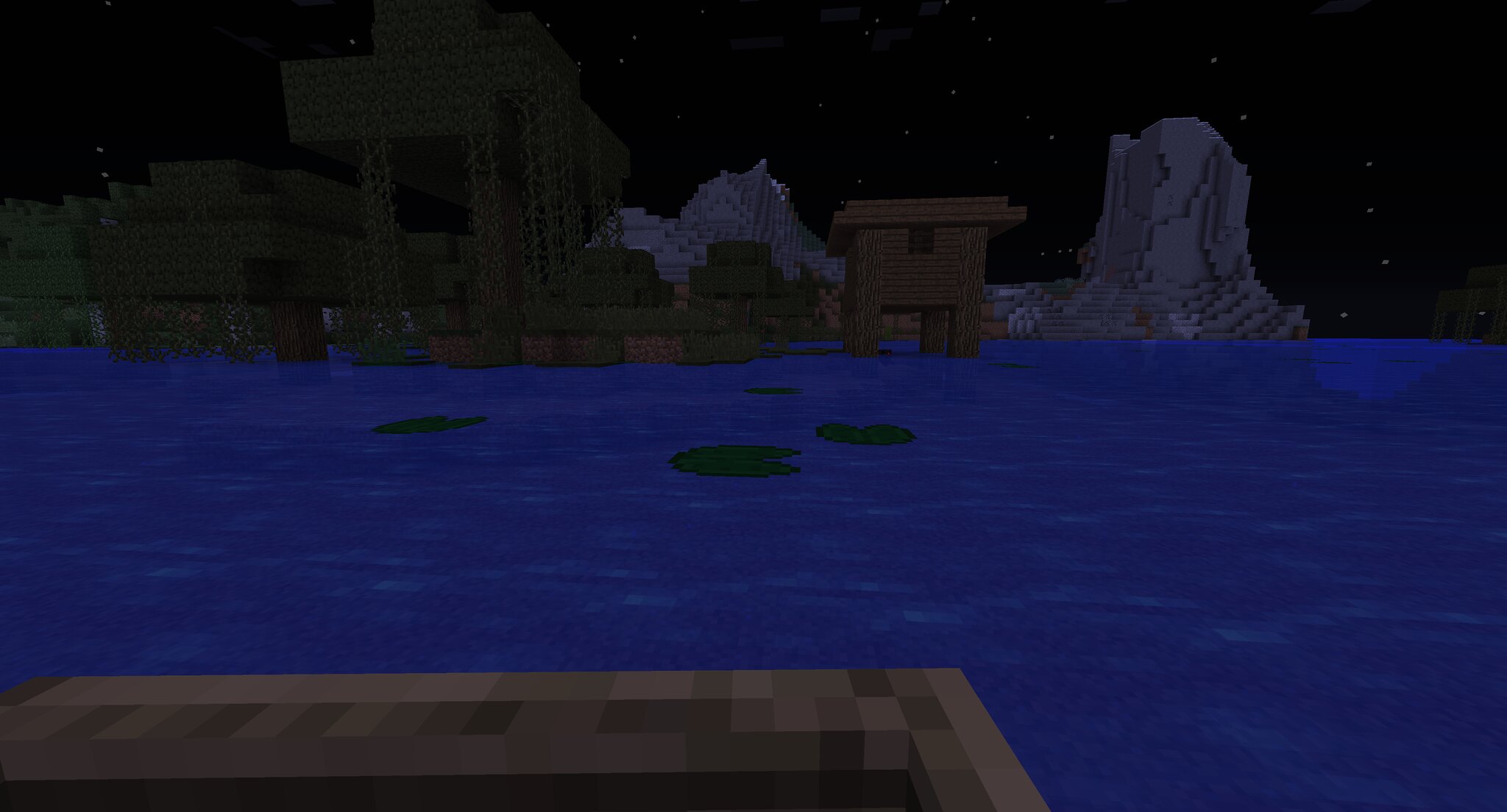A nighttime screenshot from the game Minecraft showcases a serene aquatic scene. The foreground features a calm expanse of water adorned with scattered lily pads. In the background, a dense arrangement of trees draped with willow-like vines creates an enchanting, almost mystical ambiance. Amidst the water, a rustic wooden structure adds an intriguing focal point to the scene. Distant mountains loom under a sky blanketed in black, punctuated by twinkling white stars, enhancing the tranquil atmosphere. Judging by the visual perspective, the screenshot was taken from a character seated in a boat, noticeable by the boat's rim peeking into the frame at the bottom left corner. The overall composition, rendered in Minecraft's distinctive blocky pixel art style, suggests the character is gazing from the water towards the shore, immersed in the peaceful night setting.